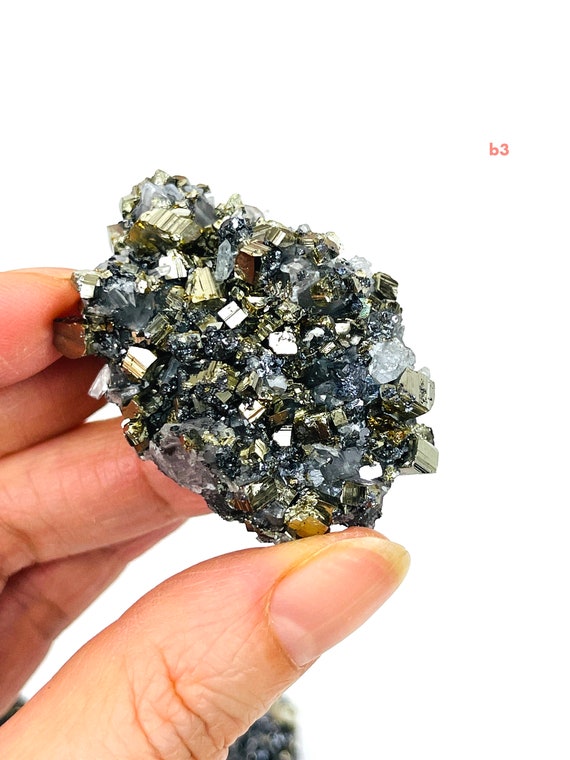A close-up image shows a polycrystalline mass held by a human hand, with visible fingers and a thumb. The specimen features cubic, gold-colored crystals of pyrite interspersed with black, silver, and clear quartz crystals, creating a clumped and angular appearance. Hints of galena or lead sulfide, with notable defects, can also be seen. The background is plain white, emphasizing the rock's intricate details. In the upper right-hand corner, there is the text "B3." The hand, belonging to a person with slightly long fingernails of indeterminate gender, securely holds this complex and shiny mineral assembly, showcasing its striking beauty and varied textures.